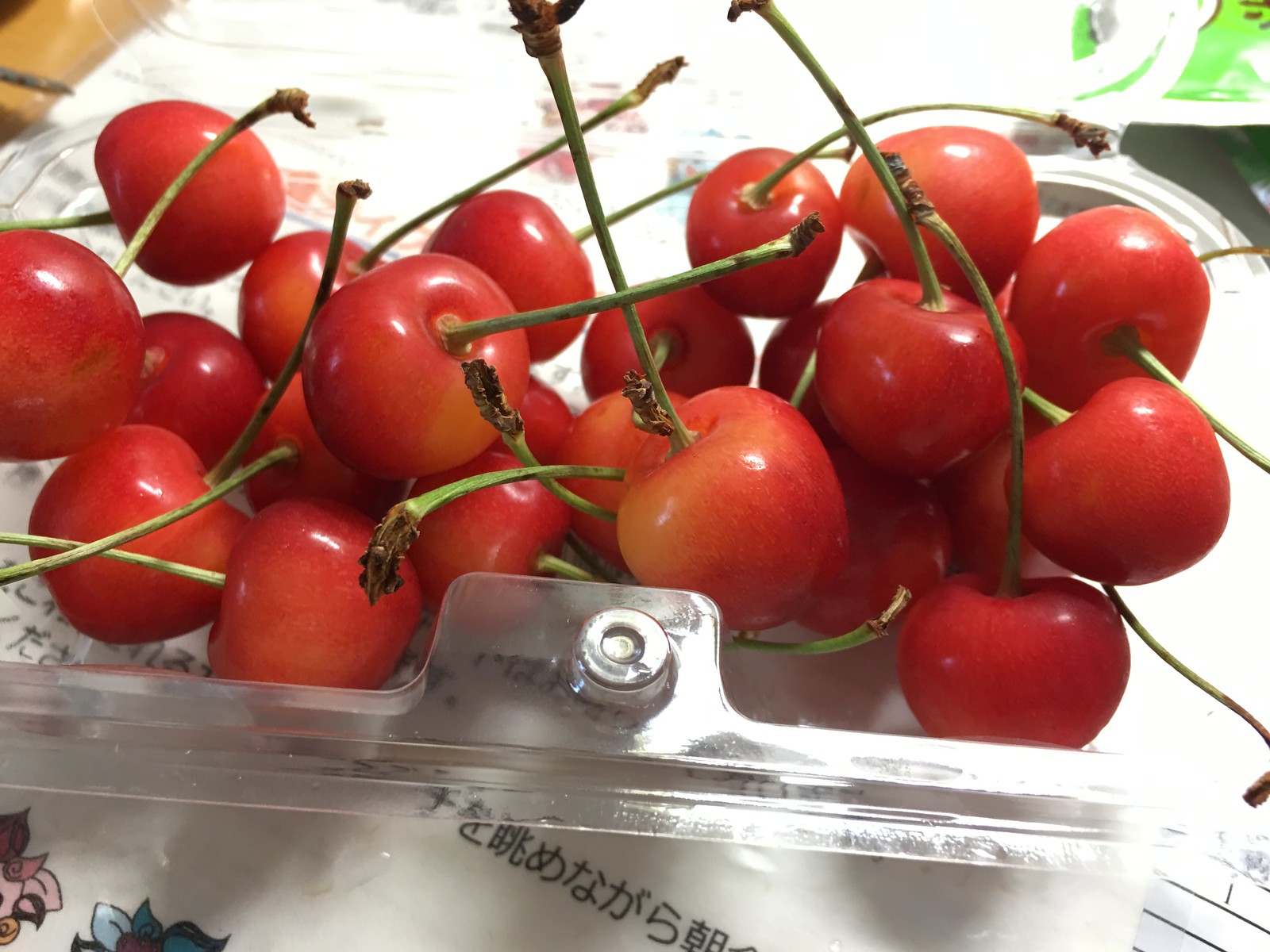The image displays a close-up view of red cherry tomatoes nestled in an open plastic clamshell container. Approximately 20 cherry tomatoes are clustered together, showcasing vivid red hues with slight orange tints and light bruising on a few. Each cherry tomato is adorned with a cute little green stem, some of which show signs of browning at the top. The transparent container sits atop a piece of paper embellished with sketches of a pink and a blue flower, along with writing in what appears to be Chinese characters. In the upper right corner of the image, a splash of lime green color is noticeable, while the upper left corner features hints of yellowish-brown.